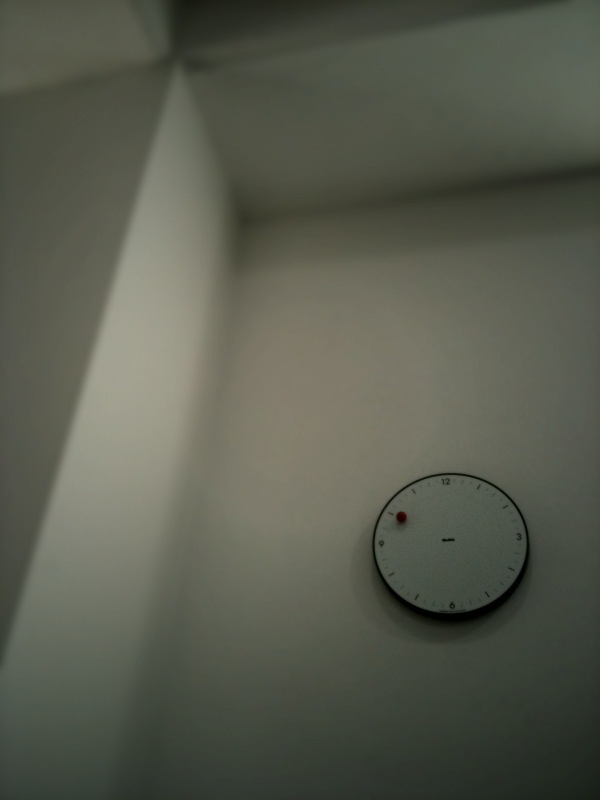The image is a vertical shot taken from a low vantage point, looking up toward the ceiling of an interior space. On the left side of the image, there are visible vertical structures which seem to be air ducts running alongside the wall. The photograph is notably blurry, creating a somewhat indistinct view. Dominating the right-hand side of the frame, below the midpoint, is a wall-mounted clock. The clock features a classic design with a black ring encircling a white face. Numerals for 12, 3, 6, and 9 are clearly marked, along with additional markers for the other hours. A distinct red circle is present on the clock face, possibly as part of the design or indicating either the minute or hour. The bottom of the image is partially shaded, which might come from an out-of-frame object casting a shadow. The walls surrounding the clock are otherwise bare, emphasizing the simplicity of the space.